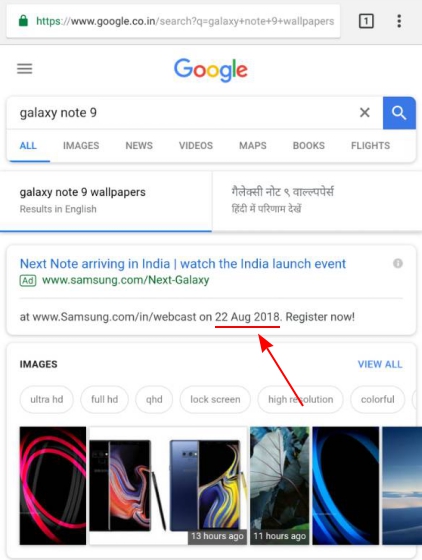The image showcases a screenshot of a Google search results page, specifically focusing on the search for "Galaxy Note 9." At the top center of the image is the URL, which reads "www.google.co.in," indicating the Indian version of Google. Adjacent to the URL is a green padlock icon and green "HTTPS," signifying a secure connection. To the far right, there is a square box with the number "1" and a vertical stack of three dots, likely indicating a menu or options button.

Dominating the top-center of the page is the colorful Google logo, with its letters in the familiar blue, red, yellow, green, and red sequence. To the left of the logo is a hamburger menu icon. Below the Google logo lies the search bar displaying the query "Galaxy Note 9." Underneath the search bar, there are several categories for further refining the search: All, Images, News, Videos, Maps, Books, and Flights.

The search results start with the phrase "Galaxy Note 9 wallpapers," followed by a grid of images depicting various wallpapers for the Galaxy Note 9. Among these images, notable mentions include a red Galaxy Note 9 phone and a blue one positioned towards the bottom right of the image.